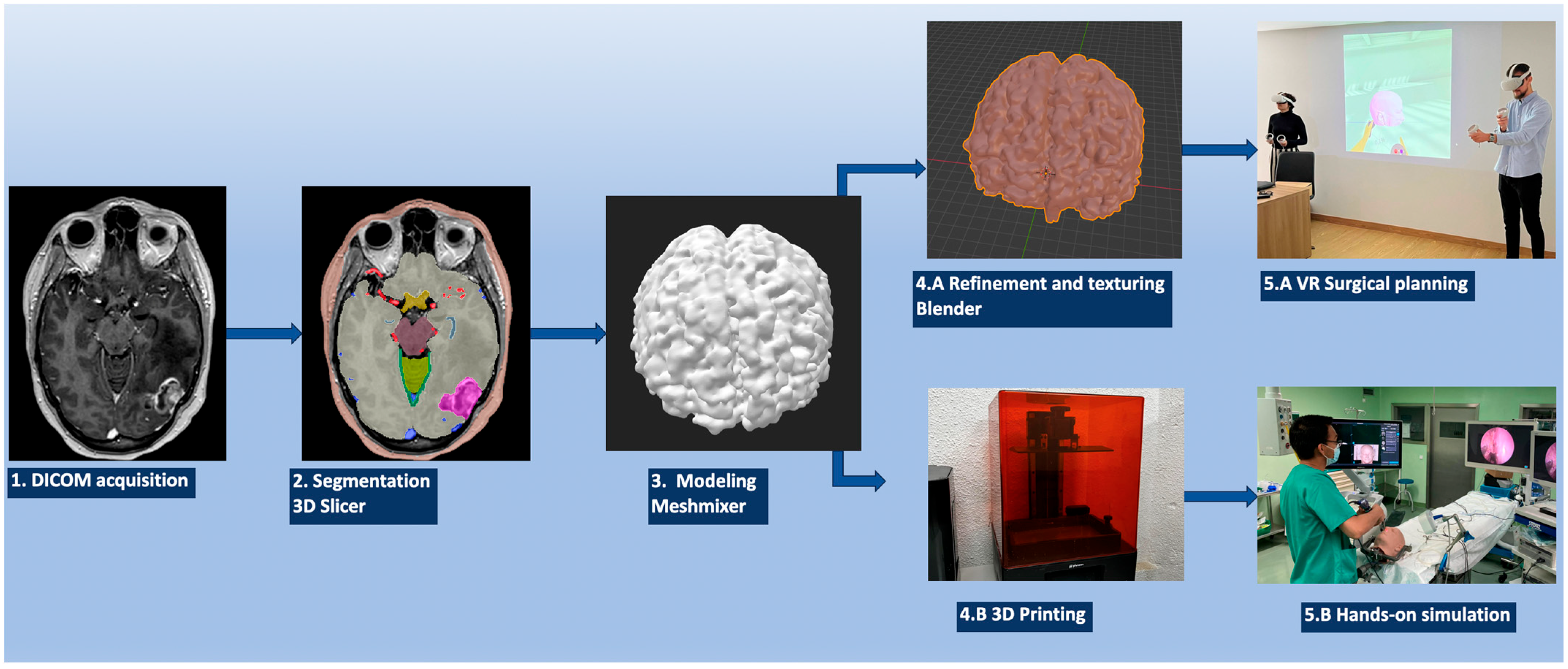The rectangular image, approximately six inches wide and two inches tall, features a series of interconnected medical infographic photographs set against a blue background that transitions to a lighter blue towards the top. The arrangement comprises seven small square photos divided into two main sections: the left section with three photos side-by-side, and the right section with two rows, each containing two photos.

1. The first image on the left, labeled "1. DICOM Acquisition," shows a black and white x-ray scan of a brain, identifiable by the visible eyeball sockets.
2. The second image, "2. Segmentation 3D Slicer," depicts the same brain scan, enhanced with various colors to highlight different areas.
3. The third image, "3. Modeling Mesh Mixer," showcases a white model of the brain with a black background. Arrows extend from this model to the top and bottom photos on the right.
   
   - Top row:
     1. The left photo, "4A. Refinement and Texturing Blender," portrays a brain model in a reddish-peach hue.
     2. The right photo, "5A. VR Surgical Planning," features two people, one in a black shirt and the other in a light blue button-down, both wearing VR headsets. They are positioned in front of a screen, suggesting they are engaged in a VR-assisted surgical planning session.
   
   - Bottom row:
     1. The left photo, "4B. 3D Printing," displays a 3D printer housed in a red case.
     2. The right photo, "5B. Hands-On Simulation," shows a doctor in green scrubs practicing a procedure on a dummy in a surgical room.

Arrows between these labeled images convey a sequential process, emphasizing the application of various technologies in medical imaging, modeling, virtual planning, and simulation.